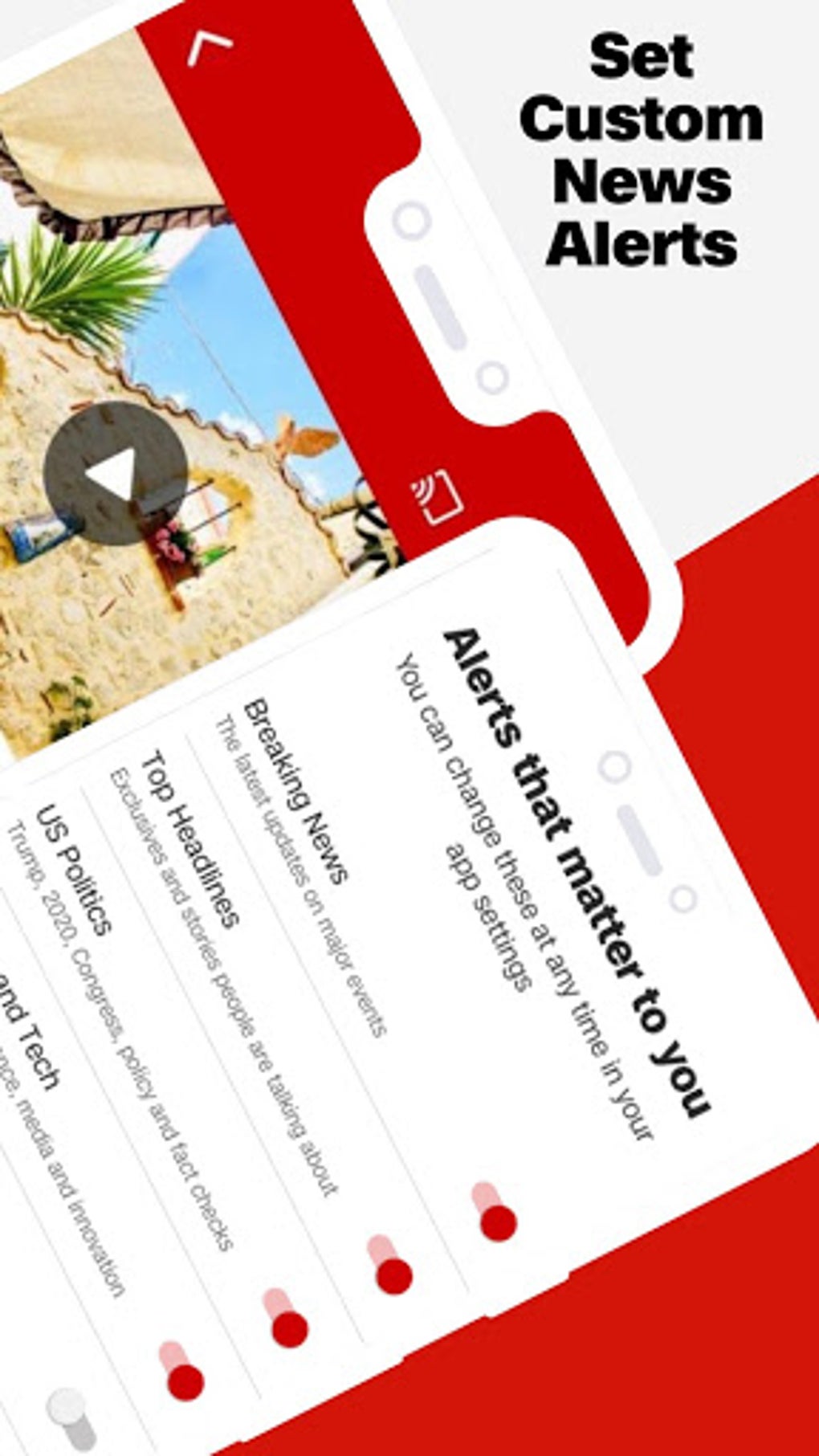The image is a screen capture, likely intended for an advertisement. At the top of the image, a simulated white cell phone with a large white notch is prominently displayed. This notch features two gray circles. On the phone screen, a red banner with a white back arrow and a white screencast icon is visible. Below this banner, a gray-and-white play button appears over a nature scene that includes a vivid blue sky, a green tree, a tan stone structure with a window, and some plant life.

Above the phone, black text on a gray background reads: "Set custom news alerts." Below the phone, a red triangular shape draws attention to another simulated white cell phone, distinguished by a thin gray line and two circles similar to those on the first phone. This phone's screen features text on a white and black background, stating: "Alerts that matter to you. You can change these at any time in your app settings."

The phone lists several types of alerts, each accompanied by a red circle:
1. "Breaking news: The latest updates on major events."
2. "Top headlines: Exclusives and stories people are talking about."
3. "US politics: Trump 2020, Congress policy, and fact checks."
4. A partially visible fourth alert mentions "tech," "media," and "innovation."

At the bottom of the screen, a gray circle is present.